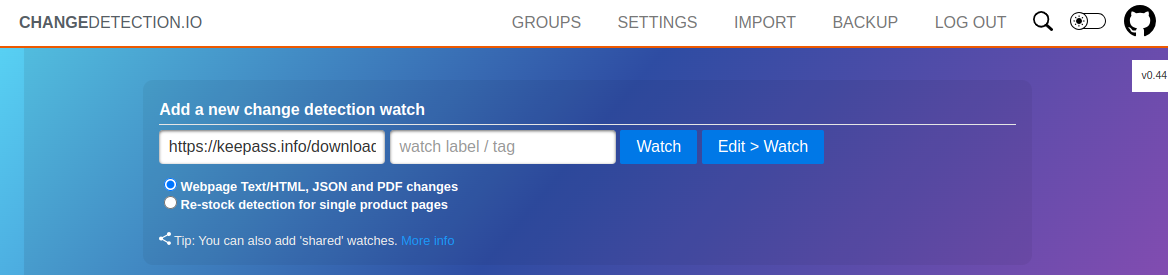**Descriptive Caption:**

This image illustrates a section of a web page dedicated to "Change Detection," though the heading could be interpreted as "Change Detection IQ" or "Change Detection IO" due to its unclear formatting. The top of the page features a navigation bar with options: "Groups," "Settings," "Import," "Backup," and "Logout." On the extreme right of the navigation bar, there's a small round button with the outline of a cat icon.

Below the navigation bar, within a blue rectangular section, there's a selection panel titled "Add a New Change Detection Watch." This panel includes an input field pre-filled with "https://keypath.infold/download," indicating where users can enter URLs for monitoring. Users have options to "Watch," "Edit," or set another "Watch."

A checkbox is ticked for monitoring "Web Page Text, JSON, and PDF changes." Another monitoring option available is "Restock Detection for Single Product Pages." At the bottom, there's a tip informing users that they can "also add shared watches" with a link for "more info."

This detailed interface suggests a robust platform for tracking changes on specified web pages, with user-friendly features for customization and various types of content monitoring.